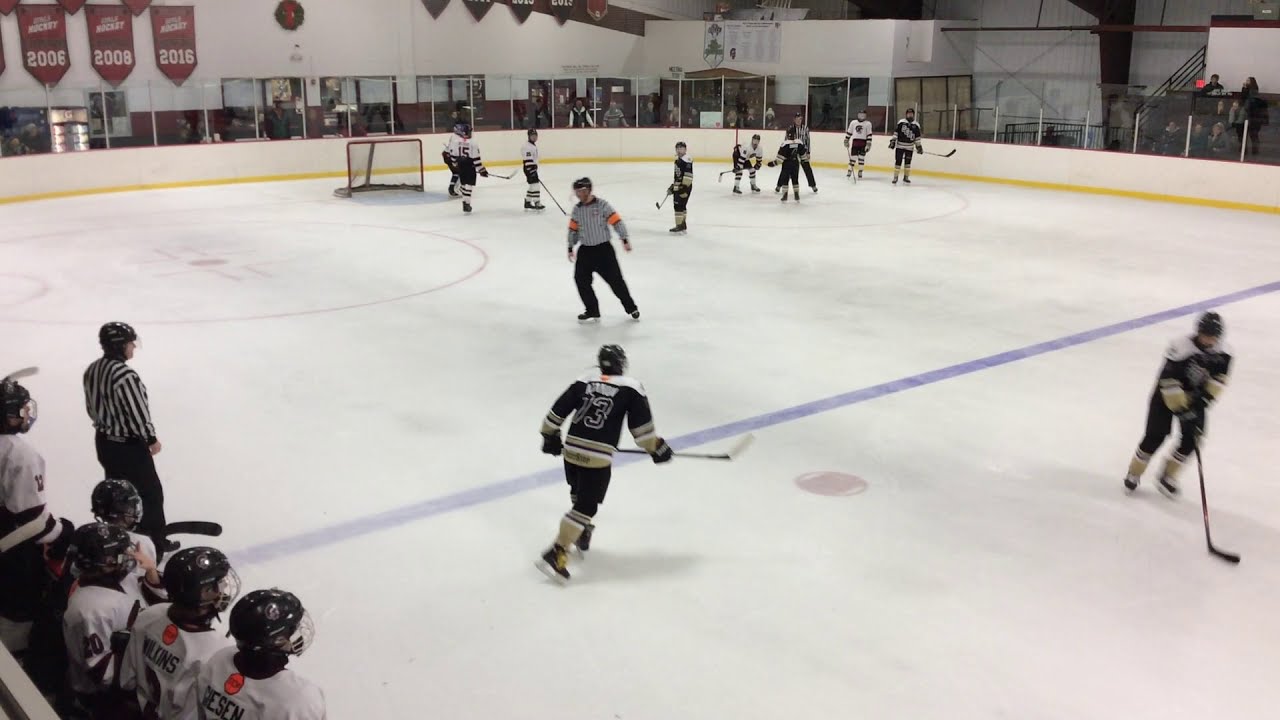This photograph captures a dynamic moment in an ice hockey stadium where a lively game is in progress. The scene is set on a white ice rink patterned with blue stripes and red goals, along with red dots marking specific spots on the ice. In the thick of the action, we see players from two teams, one dressed in black and white shirts paired with black shorts, and the other in white shirts and black shorts. The players are equipped with hockey sticks, some of them skating, others in various stages of motion or standing. Two referees, clad in black and white stripes, are on the rink managing the game.

On the sidelines, there are alternate players in orange, white, and black jerseys, sitting with their backs to the camera, waiting for their turn. The rink is enclosed by a partition that runs all the way around, with spectators intently watching the match from different elevations in the stadium seating area. In the background, the white walls of the stadium are adorned with posters or championship banners displaying the years 2006, 2008, and 2016, positioned on the upper left side. The walls also feature numerous doors, along with entryways leading into the rink area. The entire atmosphere is charged with the energy of the game and the anticipation of the spectators.